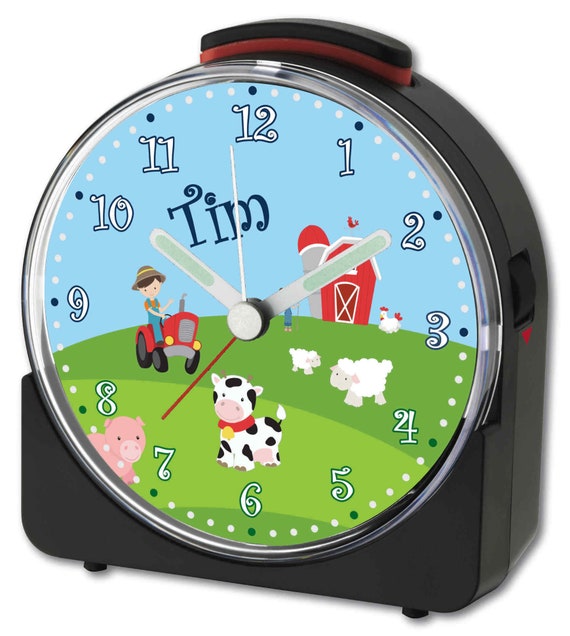This is a color close-up of a child's analog alarm clock with a black base and sides made of black plastic. The clock face features a cartoon-style farm scene with a green hill and blue sky, and has the name "Tim" written on it. Central to the image is a boy driving a red tractor. The farm background includes a little red barn with a rooster atop it, and another person standing near the barn. Additional animals in the scene include a cow with a red collar and gold bell, a pig, and two sheep—one adult and one baby lamb. The clock face is marked with numbers 1 through 12 in stylized lettering, and it has four hands: a small gray one, a larger gray one with strips of green, a thin white one, and a thin red one, currently pointing to roughly 10:10. There are also a large button at the top for stopping the alarm and a dial on the right-hand side. The base includes small dots to prevent scratching. Overall, the clock exudes a playful, childlike charm with its vivid and engaging farmyard illustration.